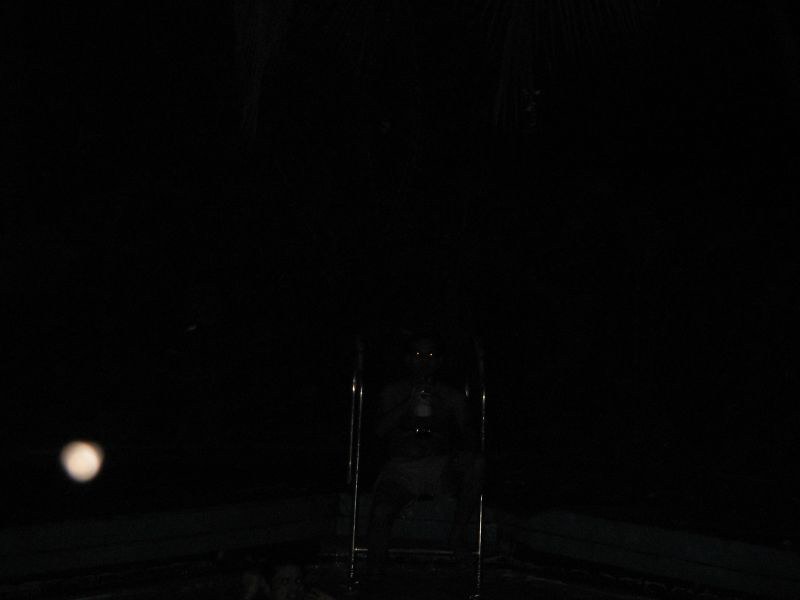This rectangular, horizontal photograph, taken at night, captures an almost pitch-black scene with a haunting atmosphere. The central focus is a dark, humanoid figure, which appears to be a robot or eerie entity, seated in what is either a shiny chair or walker. The figure has reflective, bead-like eyes that seem to stare back at the viewer, adding to the unsettling feel of the image. Light gray and silver accents highlight parts of the figure's torso and legs, as well as the rails of the chair or walker. Toward the lower left of the image, there is a hazy, tanned circle with a white center, reminiscent of an orb or the moon, adding a surreal touch. The photograph's backdrop is entirely black, intensifying the mysterious and ghostly ambiance. The reflective surfaces and glowing eyes are the only elements piercing through the darkness, creating a sense of a sinister presence lurking within the frame.